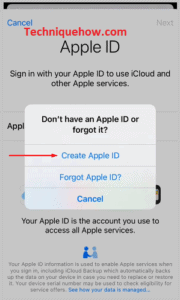The image appears to be a screenshot of a website page, primarily greyed out with a prominent white pop-up box situated at its center. At the top of the screenshot, a thin black edge is visible. The text throughout the screenshot is notably blurry, hindering full legibility. Despite this, the word "Summit" is distinguishable in a larger font, although the user feels the need to open a new tab and zoom in for better clarity, typical of their usual process as iterated by their recurring phrase, "just bear with me." 

Upon zooming in to approximately 300%, the user identifies several elements. In the top left corner, there is the word "Cancel" in blue and the domain "techniquehow.com" in red, which may appear overlaid. In the upper right corner, the word "Next" is visible in grey. The central portion of the pop-up features "Apple ID" in black text, followed by the prompt, "Sign in with your Apple ID to use iCloud and other Apple services." 

Additionally, within the pop-up, there's a highlighted section stating, "Don't have an Apple ID or forgot it?" accompanied by a red arrow pointing towards the options. Below this, options such as "Create Apple ID" in blue and "Forgot Apple ID" and "Cancel" are noted. The bottom section of the pop-up contains the statement, "Your Apple ID is the account you use to access all Apple services," and an infographic depicting two blue figures shaking hands. 

Despite zooming, some grey text underneath remains illegible, with a snippet of blue text discernible at the bottom. The overall grey-out of the image contrasts with the white pop-up box, enhancing its prominence yet contributing to the peculiar visual appearance.